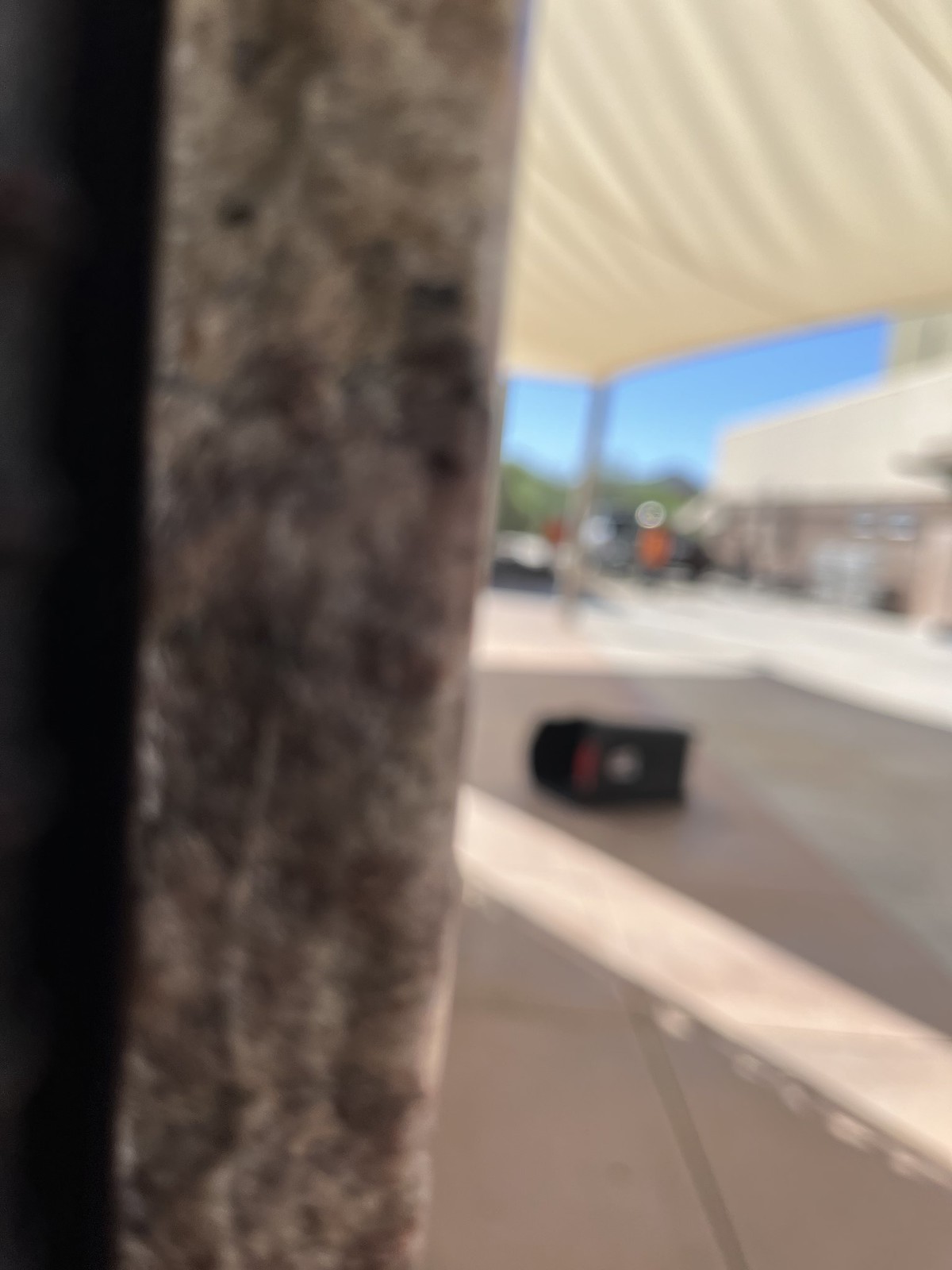The photograph presents a blurred outdoor scene featuring a stony, textured concrete wall or pillar on the left side, marked by gray and black hues. Adjacent to it is a dark, vertical strip. The image's right side reveals a concrete floor partially shaded by an overhead beige cloth awning with a distinct rippling pattern, casting a shadow underneath. A black object, possibly a piece of luggage or a chair, lies near the center bottom of the image. In the distance, blurred shapes suggest parked vehicles and a white tent top is visible in the upper right corner. The background showcases faintly visible green hills and beige rectangular structures, under a clear blue sky.